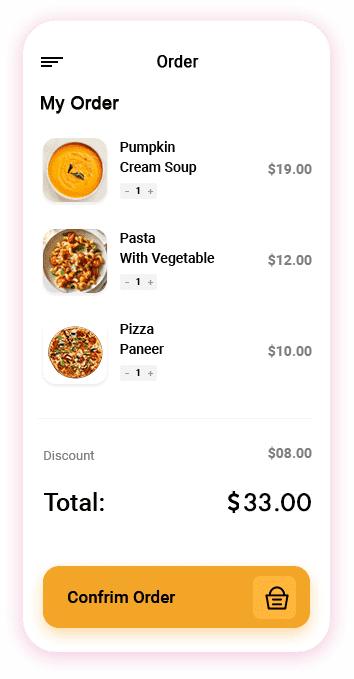The image is a screenshot of a cell phone displaying a food delivery app. The background is predominantly white, and the page is labeled "Order," centered at the top. To the left of the title "Order" is an icon consisting of three vertically stacked lines, each progressively shorter than the one above.

Below the top bar, bold text reads "My Order," followed by three listed items. The first item is a bowl of orange soup, identified as "Pumpkin Cream Soup" costing $19, with one bowl selected. The next item is "Pasta with Vegetables" priced at $12, accompanied by an image of the dish. The final item is "Pizza Paneer" for $10, also with one selected, featuring a picture of the pizza. Each image is enclosed in a rounded square frame.

Beneath the listed items, the text "Discount $8" is displayed, leading to a bold total of $33. The words "Total" and "$33" are in larger font compared to the rest of the text on the page.

At the bottom is an orange, rounded rectangular button with the misspelled text "Confrim Order." Next to it is a slightly lighter, rounded square button containing an icon that could either be a lock or a shopping basket.